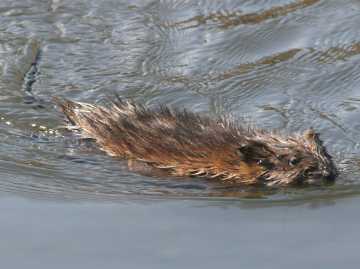This image captures a compelling nature scene of an animal swimming through water, which is likely a beaver, though it could also be a muskrat due to the lack of tail visibility. The animal is positioned centrally and is swimming towards the right-hand side of the frame. Its fur, a blend of brown and reddish-brown shades, is slicked back from the water, with a grayish tint on the front of its face. Its black eyes and nose are noticeable, giving a clear look at its facial features. The water surrounding the animal is a murky brownish-gray, suggesting it could be from a lake or possibly floodwater. The surface of the water is relatively calm at the bottom of the image, but there is a noticeable wake created by the animal's movement in the top two-thirds, enhancing the sense of motion. The tail of the animal is not visible, likely submerged.